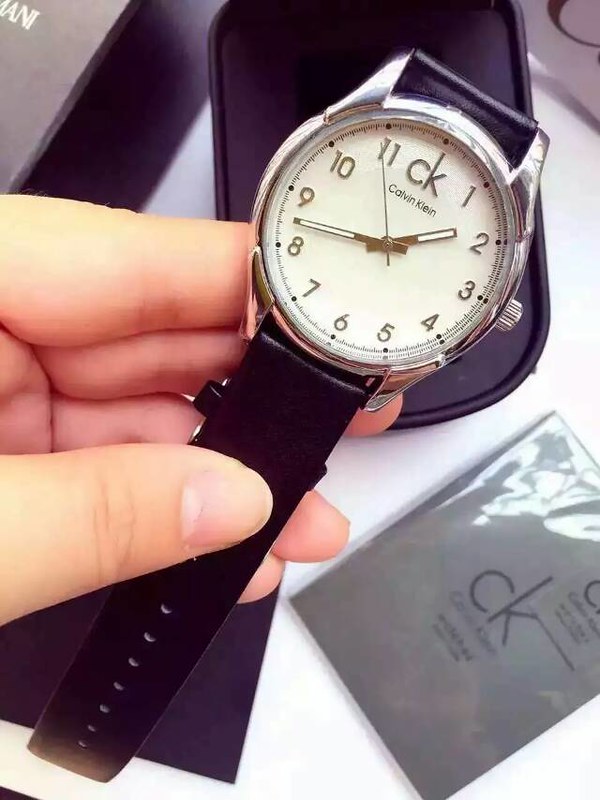This image features a stylish Calvin Klein watch prominently displayed. The watch boasts a sleek black leather band that angles down towards the lower left corner of the frame. Its silver face, positioned towards the upper right corner, is adorned with luminous hour, minute, and second hands, making it easy to read in the dark. The analog display is elegantly simple, featuring the CK logo in black below the 12 o'clock position, and markers for each hour from 1 through 11. The current time displayed is 1:42 and 54 seconds. The watch includes a silver stem for winding, which is visible on the side.

The watch is being held by a left hand; the thumb secures the band while two fingers are placed underneath the watch face and the other two beneath the band. Beneath the watch, there is a black case, and in the bottom right corner of the image, a gray package labeled "CK Calvin Klein" is partially visible. A mysterious black object can also be seen in the bottom right area. The entire arrangement is set on a white table, with some gray shading around the edges.